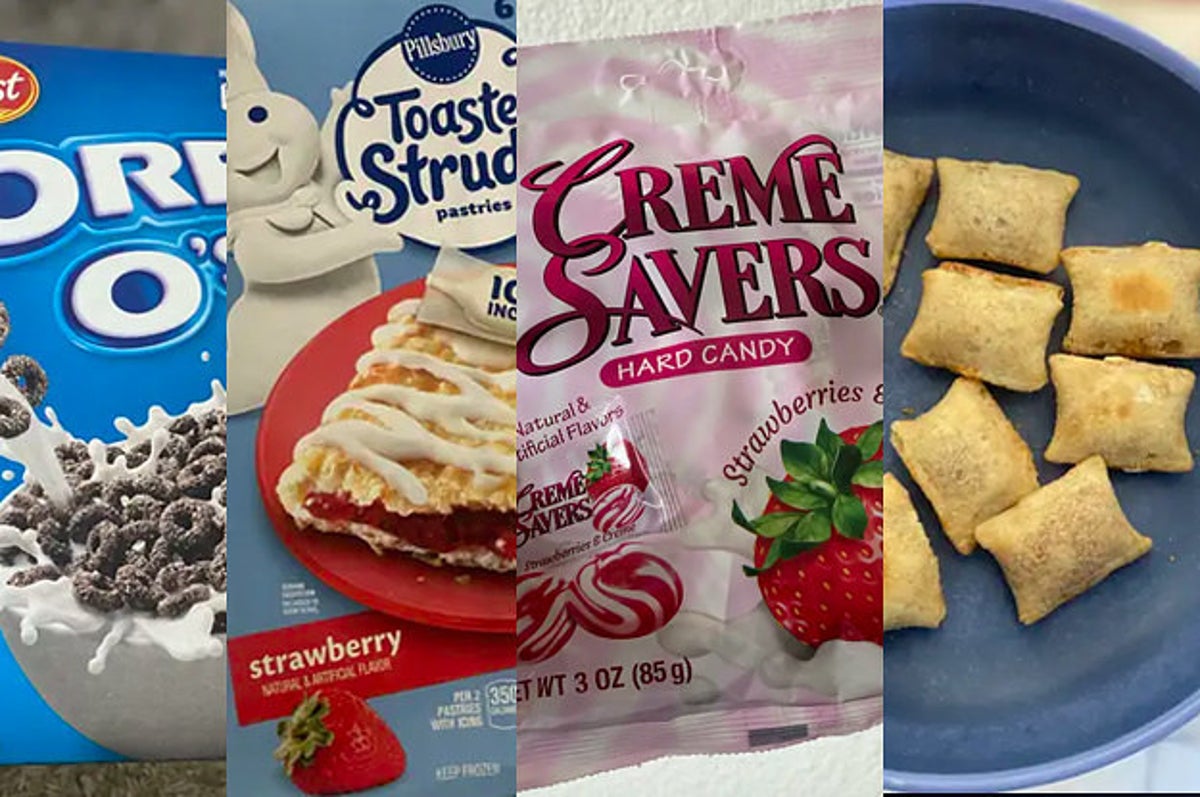This horizontally aligned rectangular image is divided into four vertical slices, each showcasing a different food item. 

On the far left, there's a partial view of a box of Post Oreo O's cereal, featuring a prominent "O" from the word "Oreo" and a bowl filled with milk and round chocolate cereal pieces resembling mini Oreos. 

Next to it, the second slice highlights a Pillsbury Toaster Strudel box, predominantly showcasing the Pillsbury Doughboy and the words "Toaster Strudel" in blue. The focus is on a strawberry-flavored strudel, depicted with a filling of strawberries and topped with icing, laid out on a red plate.

The third section features a package of Cream Savers Hard Candy in strawberry flavor, illustrating candies with red and vanilla swirls alongside an image of a strawberry. The package indicates it contains 3 ounces (85 grams) of candy.

On the far right, there's a blue pottery plate with several golden-brown pizza squares, likely Totino's pizza rolls, suggesting they've been cooked and ready to eat. 

Together, these strips present a variety of appetizing foods that are both nostalgic and enticing.